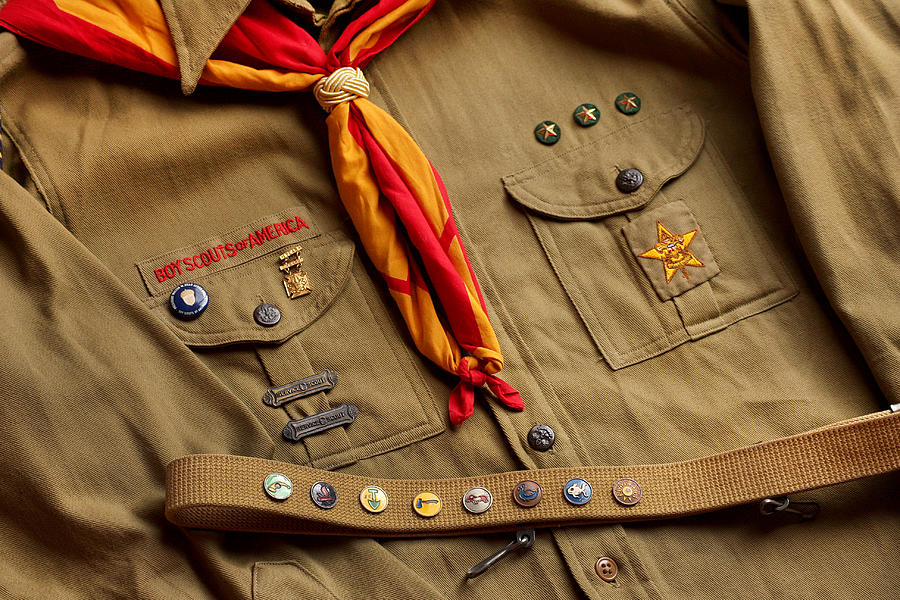This detailed photograph captures the front of a Boy Scout uniform laid flat on a surface, showcasing its intricacies predominantly from the chest down to the waist. The uniform features a brown button-up shirt with folded sleeves, two chest pockets with dark buttons, and a red and yellow neckerchief tied around the collar. 

On the left chest pocket, there's an embroidered patch that reads 'Boy Scouts of America' in red thread. Just above this pocket, there’s a blue pin featuring an acorn and to its right, a golden pin. The pocket fold also has two brass-colored horizontal bars attached.

On the right chest pocket, three gold stars in black circles are pinned above it, alongside a sewn-in Boy Scout star emblem. Draped across the uniform is a sash adorned with a series of merit badges showcasing various icons such as a sun, a fish, a duck, a dog, an axe, and a shovel, with some badges indistinct. This nuanced presentation highlights the meticulous details and symbols of accomplishments and affiliations in the Boy Scout uniform.